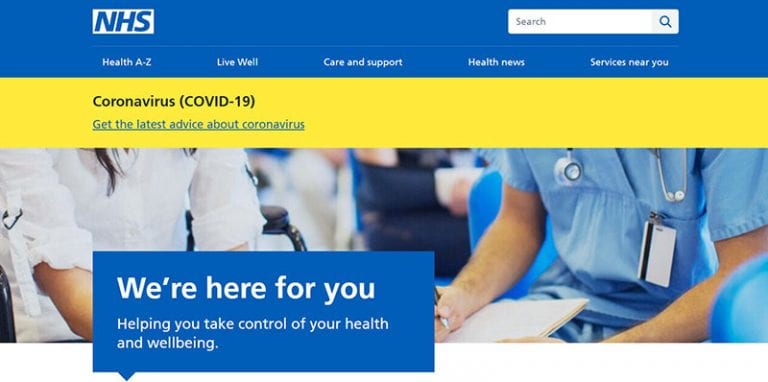The image is a screenshot of a website featuring a prominent blue banner at the top. Inside the banner, slightly offset from the left, is a white rectangle with the capitalized letters "NHS" prominently displayed. To the right of this, there is a white search bar with a small gray square containing a magnifying glass icon.

Below the blue banner, white text spans across the page offering navigation options: "Health A to Z," "Live Well," "Care and Support," "Health News," and "Services Near You." 

Further down, a bright yellow banner with bold black text announces "Coronavirus (COVID-19)" followed by a blue hyperlink urging users to "get the latest advice about coronavirus."

Beneath this, a graphic depicts medical professionals in blue scrubs and white uniforms, shown from the neck down to their waists.

A final blue banner under the graphic reads "We're here for you" in white text, followed by the statement: "Helping you take control of your health and well-being."